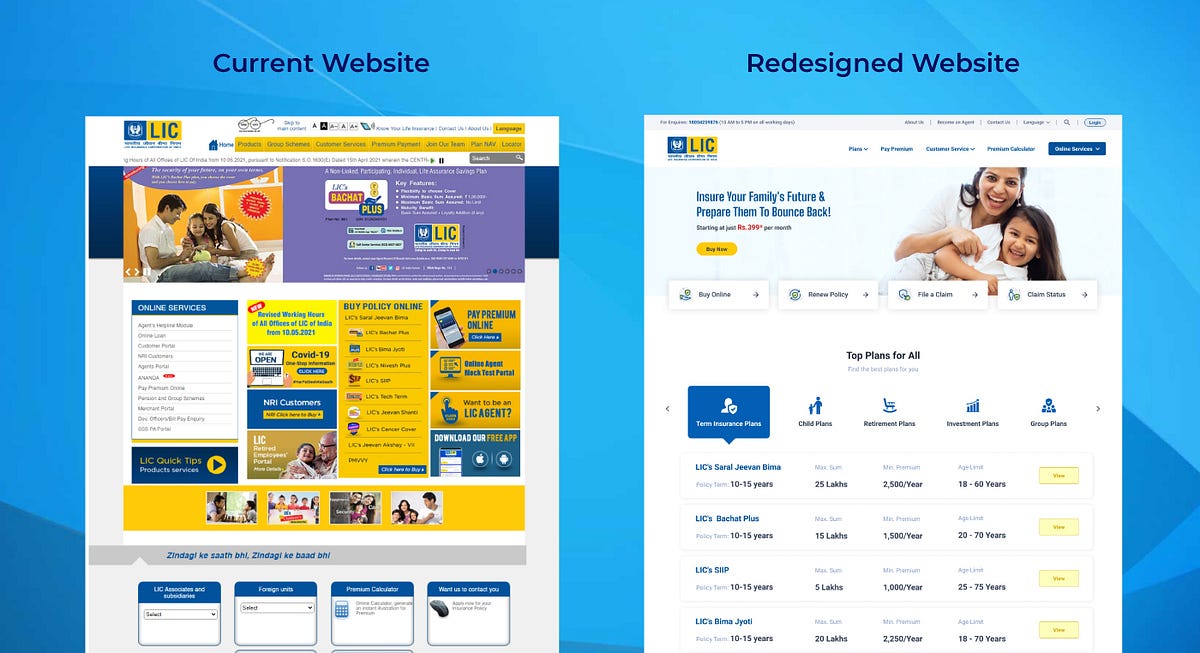Screenshot collage of the LIC website redesign. The left side displays the current website under the heading "Current Website," showcasing a cluttered and chaotic design with an overwhelming mix of bright yellow, dark yellow, blue, orange, white, and purple boxes. The visually busy and disorganized layout makes navigation challenging. On the right side, under the heading "Redesigned Website," a new screenshot demonstrates a vastly improved, clean design featuring a white background with minimal accent colors. The refined, aesthetically pleasing layout presents a user-friendly and streamlined interface, enhancing overall usability by reducing the number of boxes and clashing colors.